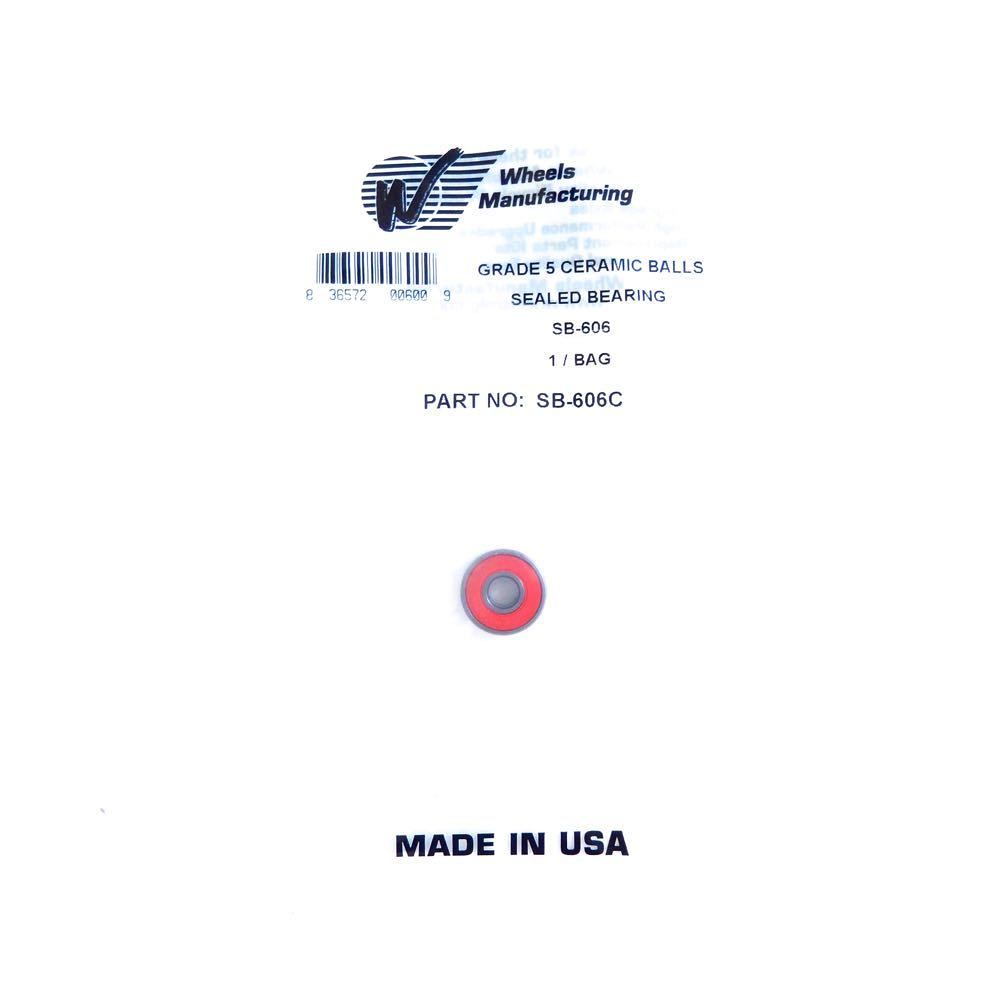The image features what appears to be a product label on a completely white background, ensuring no distractions from the primary focus of the image. At the top of the label, there is a prominent logo featuring a large "W" with the text "Wheels Manufacturing" beside it. Directly below this, there is a barcode. Under the barcode, the label reads: "Grade 5 Ceramic Balls, Sealed Bearing, SB-606, 1/Bag, Part Number: SB-606." Near the bottom section of the label, there is a red circle with a gray outline and gray center. Finally, at the very bottom of the label, in bold print, it states: "Made in USA."